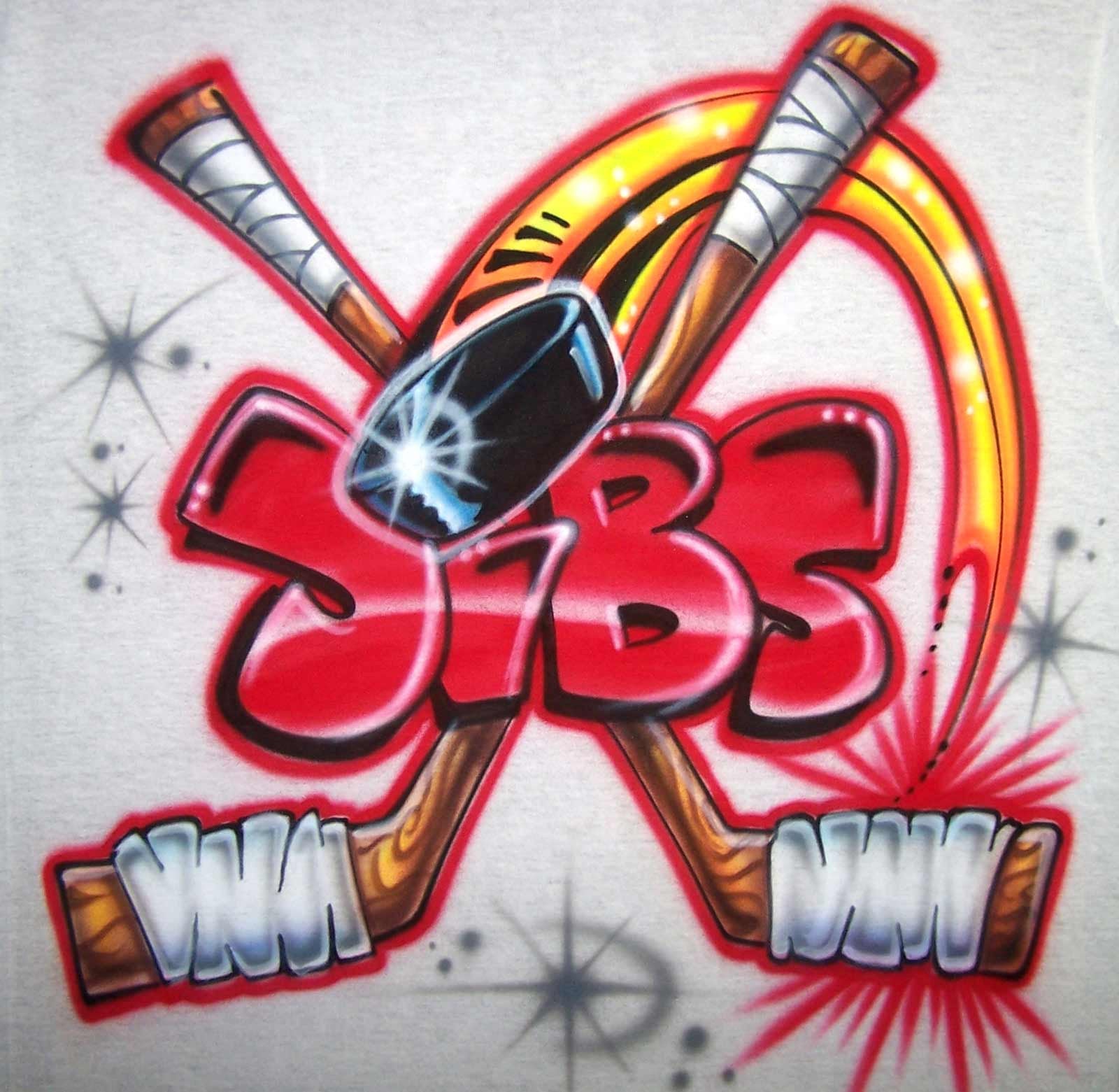This image displays a vibrant, graffiti-style design, prominently airbrushed on a white t-shirt. Central to the image are two cartoonish hockey sticks crossed in an 'X' formation, each adorned with white athletic tape around the handles and the lower parts. Highlighted in bold red paint, the design is outlined carefully, giving it a striking appearance. At the heart of the crossing sticks, the word "JIBS" is depicted in large, bubbly, red graffiti letters with heavy shadowing for a three-dimensional effect. Notably, the dot of the letter "I" is creatively replaced with a black hockey puck, which appears to be shooting forward, accentuated by dynamic yellow trails indicating motion. Surrounding the design are scattered, dark gray stars that add an extra layer of detail to this intricate piece of street art.